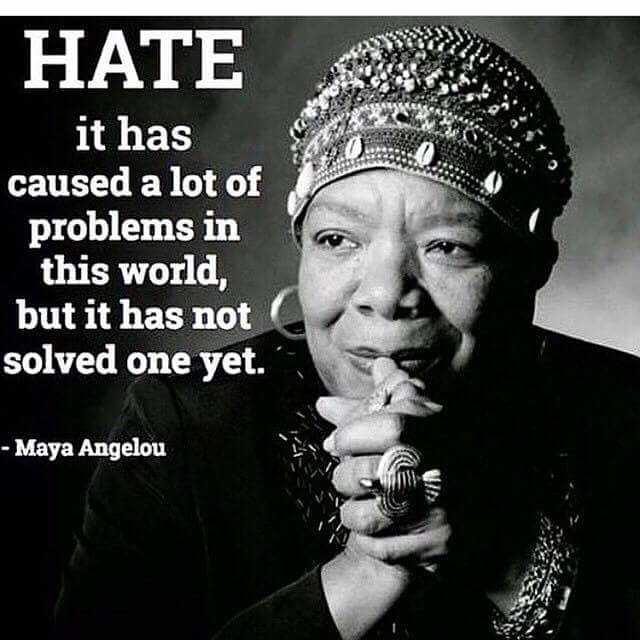The black-and-white photo features a powerful statement by Maya Angelou on the left side that reads, "HATE: It has caused a lot of problems in this world, but it has not solved one yet." The right side displays a striking image of a black woman, presumably Maya Angelou herself, staring slightly to the left. She wears a head covering adorned with an elaborate arrangement of seashells, beads, and stones of varying sizes. Her right ear is adorned with a visible hoop earring. She is dressed in a dark, long-sleeved garment and holds her hands clasped in front of her, with a prominent bird-shaped ring on one of her fingers. The background is gray, contributing to the monochromatic aesthetic of the photograph. The woman's expression carries a hint of an innocent smile, enhancing the captivating and poignant nature of the image.